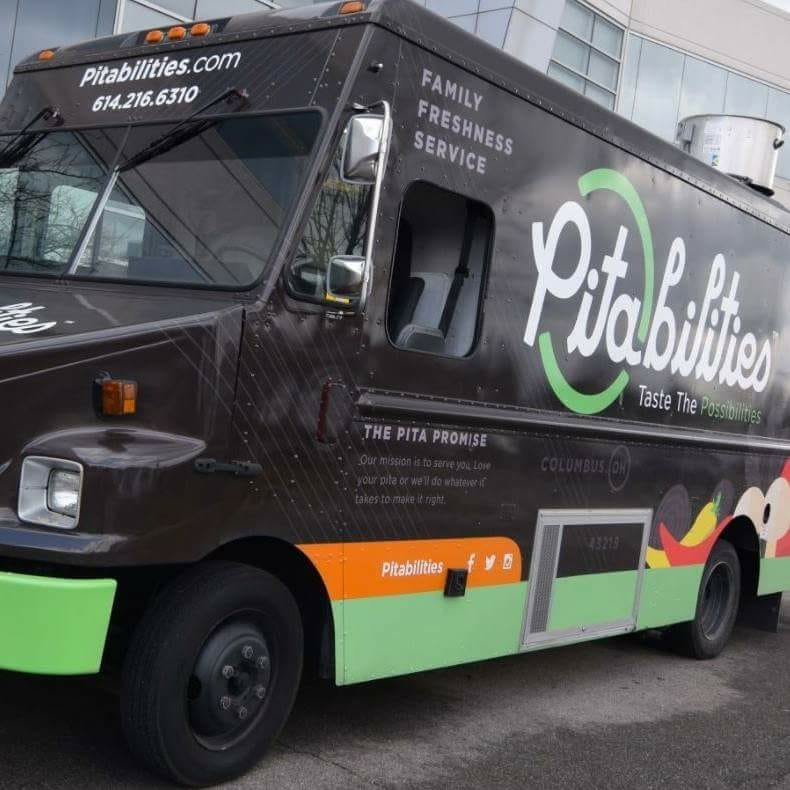This photograph features an impeccably maintained, predominantly black food truck named PETABILITIES, distinguished by a striking lime green stripe that extends from the front bumper and wraps around the bottom of the vehicle. The truck's bold branding is emphasized with a large logo on the side, where the word "PETABILITIES" is prominently displayed in white cursive font, encircled by a green circle around the letters "PETA." Below the logo, the slogan "TASTE THE POSSIBILITIES" is written in smaller text. The truck offers a visual feast with illustrations of various vegetables, including yellow and red chilies, mushrooms, and what appears to be purple onions. The front of the truck showcases the website, PETABILITIES.COM, along with a contact phone number, 614-216-6310. Additionally, social media handles for Instagram, Facebook, and Twitter are visible on the side in orange text. The setting is during the daytime with no one inside the truck. The vehicle, which might be based in Columbus, Ohio, underlines a blend of family freshness and service, potentially suggesting a connection to PETA bread products or a plant-based menu.